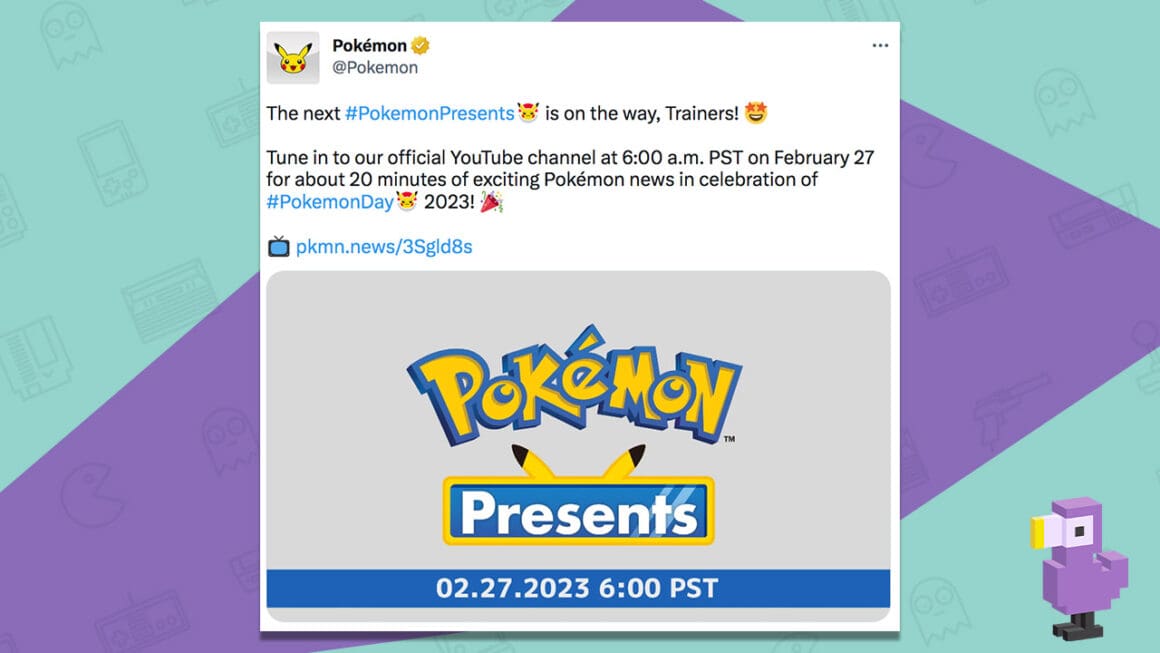The image showcases a vibrant web page dedicated to a Pokémon game. The background is predominantly a bright sky blue with an irregularly shaped purple overlay at the center. Superimposed on this backdrop is a sheer line-art drawing of various video game elements in black or gray, including a handheld Gameboy, a Gameboy controller, Pac-Man, a Pac-Man ghost, and an old-style game cartridge, blending nostalgically into the design.

Centrally, there is a white square box resembling a tweet or Facebook post. In the upper left corner of this box, a gray square houses Pikachu's character in yellow, black, white, and red colors. Next to Pikachu is a bold black text reading "Pokémon," accompanied by a gold seal featuring a white checkmark. Beneath this, the text "@Pokemon" appears in gray.

In the upper right corner of the white box is a gray ellipsis button. The post itself announces in black text: "The next #PokemonPresents is on the way, Trainers! 🌟" Below this is more detailed text: "Tune in on our official YouTube channel at 6 a.m. PST on February 27th for about 20 minutes of exciting Pokémon news in celebration of Pokémon Day 2023. 🎉" Following this is a television emoji and a blue hyperlink: "pkmn.news/3sGLDAS."

Beneath the post is a gray rounded rectangle featuring a yellow and blue Pokémon logo and a blue button outlined in yellow, with Pikachu ears protruding from the top. The button is filled with a bright blue color and bears the bold white text: "Presents." Directly under this button, within a bright blue banner, is the white text: "02.27.2023 6:00 PST."

In the bottom right corner of the blue and purple section, there is a small 8-bit style bird-like creature with a purple body, white eyes with black pupils, a yellow-tipped beak, and tiny black feet or claws. The figure has a distinctly blocky, retro video game appearance.